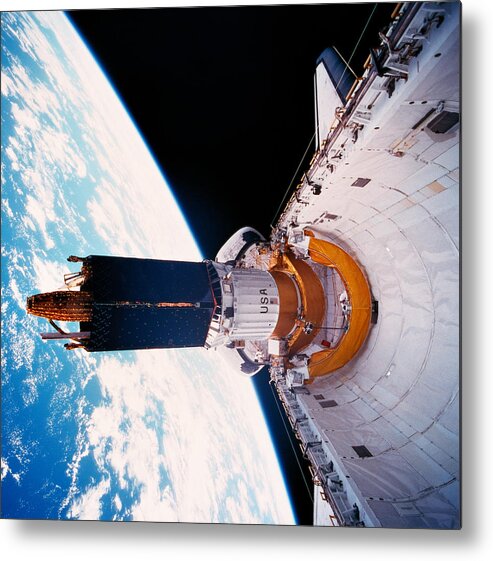The image is a color photograph in portrait orientation depicting the space shuttle floating in outer space with the Earth below. The shuttle, oriented diagonally from the right side of the image, features a triangular shape narrowing to a central point that extends into a tower structure with various arrays and black panels surrounding a central brown object. The base is painted white with corrugated metal and prominently displays the text "USA." The smokestack features some gold accents. The background showcases the vastness of space with a deep black backdrop, while the Earth appears in the lower arc of the frame, showing a diverse palette of blue, white, and brown, suggestive of oceans, clouds, and landmasses. The photo captures a realistic depiction of space with a wide view of the Earth's horizon and misty cloud formations.